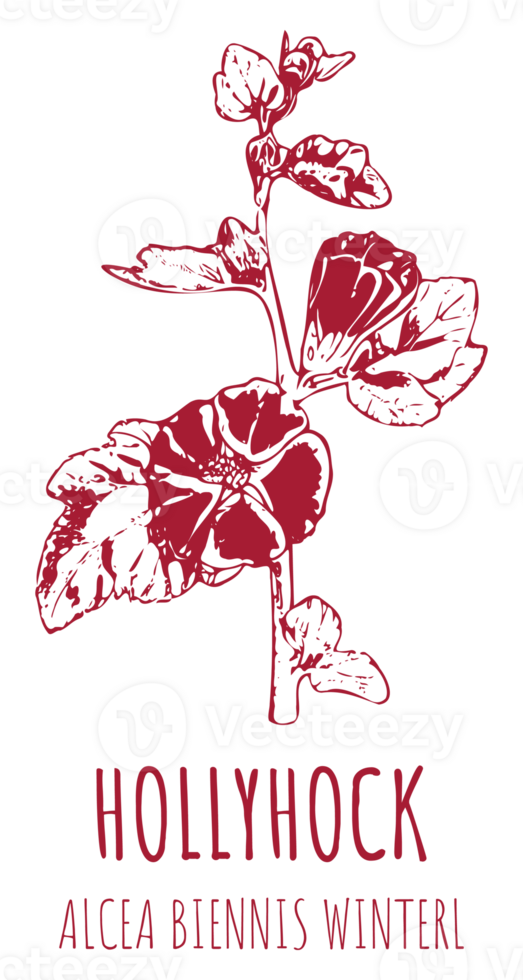This detailed print features a red ink sketch of a hollyhock plant labeled "Hollyhock" at the bottom. Beneath this, the name "Elsia Benyes Wintrell" is inscribed. The artwork, set against a white background, depicts a hollyhock with large, intricate blossoms and leaves extending from its stems. Higher on the plant, unbudded flower petals and additional foliage are illustrated. The image bears multiple Vecteezy watermarks, each featuring a distinctive V logo with a curled end, scattered across the artwork.